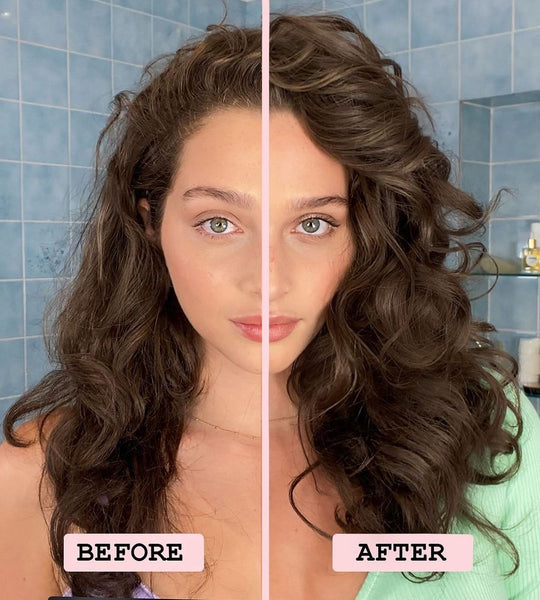The image features a before-and-after comparison of a woman in her 20s with Caucasian skin, green eyes, and dark brown, curly hair, shown in a rectangular format divided by a thin pink vertical stripe. Both photos are set in a bathroom with light blue square tiles and white grout. In the "before" image on the left, indicated by a pink horizontal rectangle with black text, the woman's hair appears flatter, duller, and matted. The "after" image on the right, labeled similarly, reveals her hair with significantly more volume, shine, and definition. Her eyes look larger and her lips slightly puffier in the after photo, while her nose appears more prominent. She wears a light mint-colored shirt and maintains a serious, no-nonsense expression in both images.